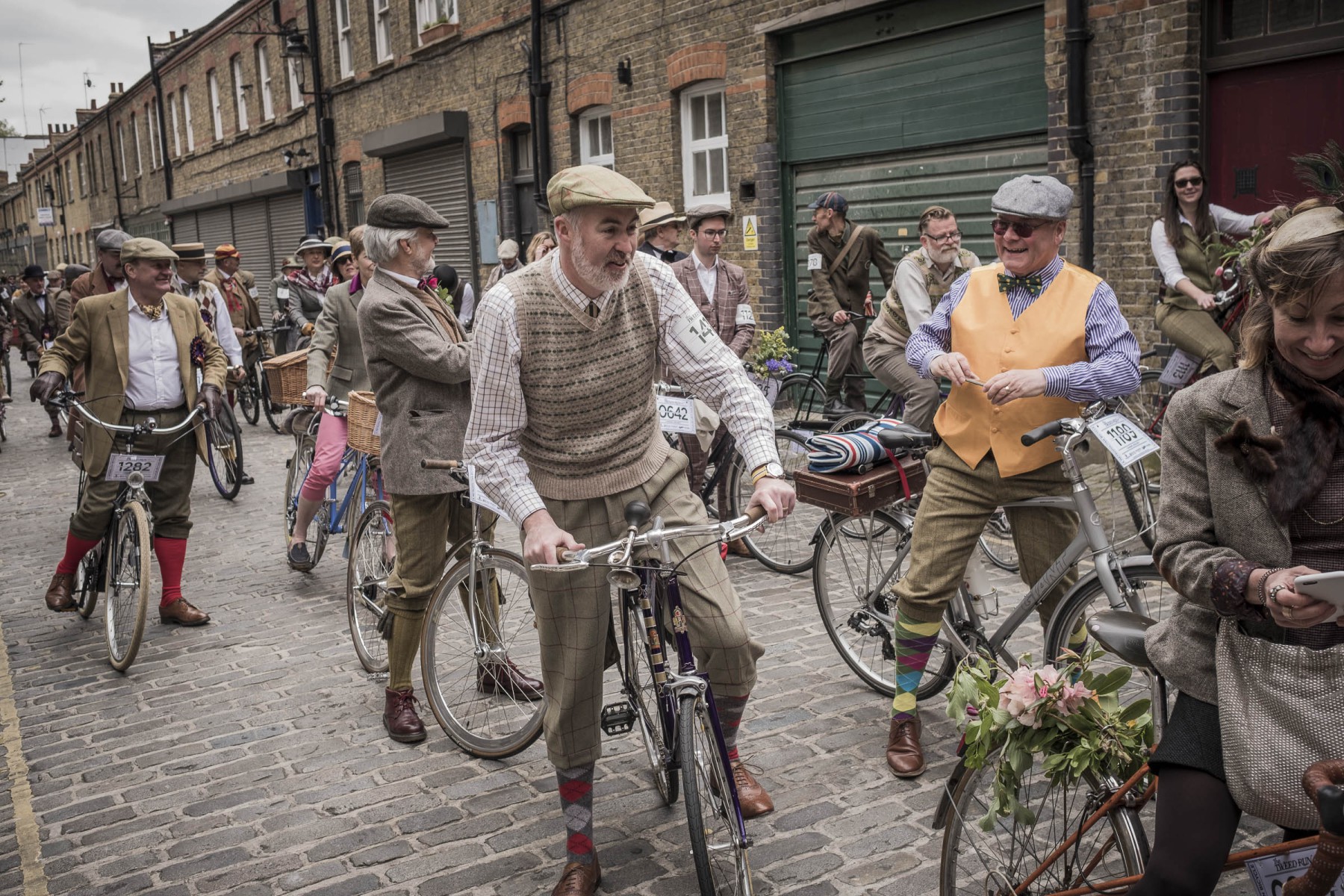The photo showcases a bustling urban scene reminiscent of the 1920s but captured in modern times. Set on a brick-paved roadway, the backdrop features a row of brick-faced buildings, each about two to three stories high with closed roll-down doors, evoking an old-world charm. The street teems with bicyclists, primarily men, who are dressed in period-appropriate attire: newsboy caps, vests, sweater vests, jackets, dress pants tucked into fancy socks, and ties. They appear in high spirits, riding bicycles that also have a vintage look. Despite the nostalgic setting, a woman at the very right foreground, holding a bag, is looking down at her smartphone, a subtle yet clear indicator of the current era. Another woman can be seen in the background to the right, leaning against a wall and wearing sunglasses. The scene appears to be a joyful gathering of sorts, with the participants immersing themselves in the historical recreation.